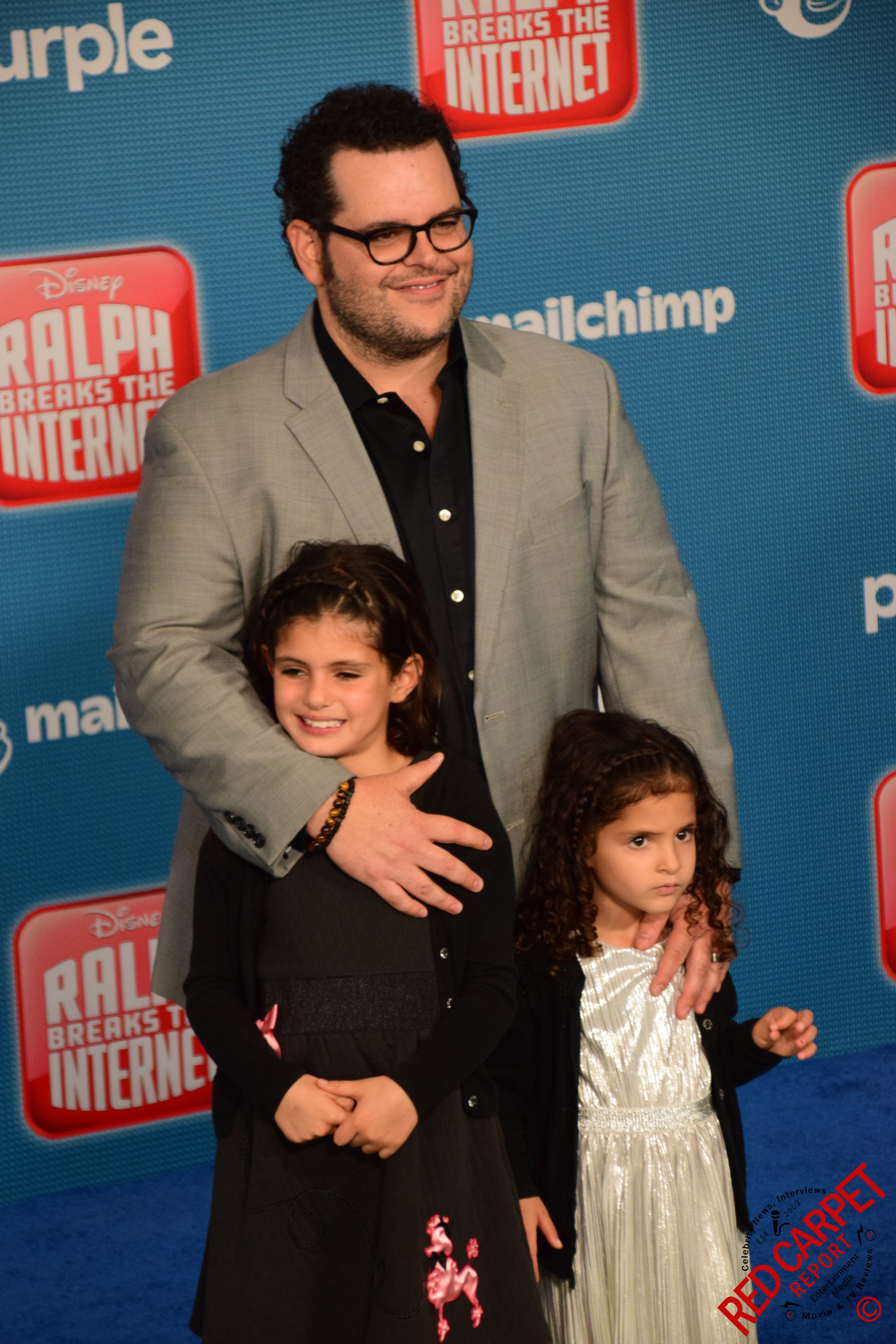The image depicts a man, possibly an actor, standing on a blue carpet at what appears to be a red carpet event for the Disney movie "Ralph Breaks the Internet," as indicated by the backdrop displaying the movie's title and logo. The man is wearing an open gray suit jacket over a black button-up shirt with white buttons. He has short, curly black hair, black-framed glasses, and a short, well-groomed beard. He is smiling and has an arm around each of the two girls beside him, who are likely his daughters. The taller girl on the left, who is smiling and showing her top teeth, is dressed in all black with a pink poodle design on her dress. The shorter girl on the right, who has a serious expression, is wearing a shiny white dress paired with a black long-sleeve open shirt. Both girls have curly, brown hair. In the backdrop, there are additional displays, including the text "Ralph Breaks the Internet," the Disney logo, the word "Mailchimp" partially visible over his right shoulder and below his left elbow, and a red square with the Disney logo positioned beneath the words "Ralph Breaks the Internet."